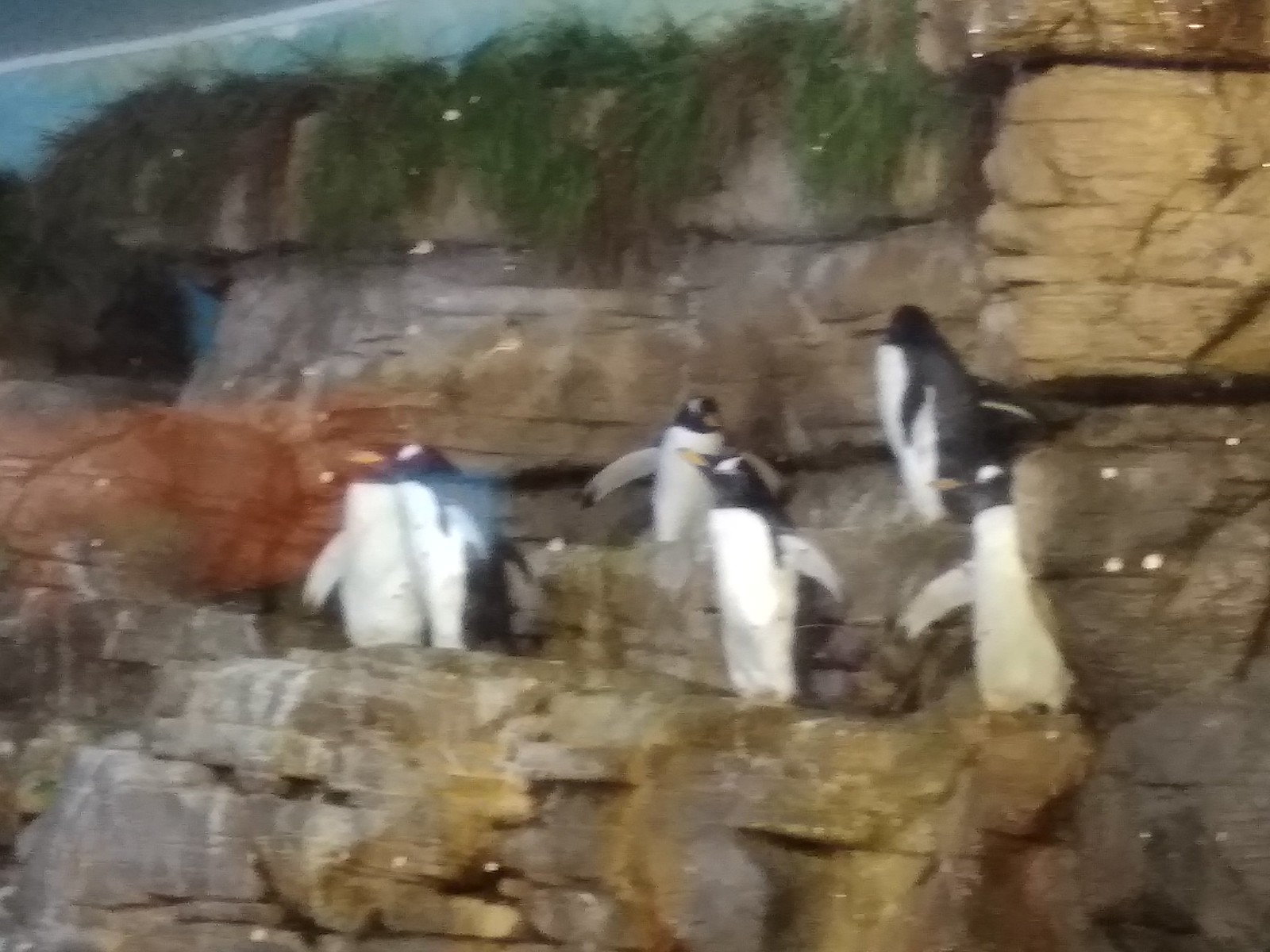This is a blurry indoor color photograph of a zoo or aquarium enclosure featuring six penguins, likely emperor penguins, standing on a realistic, staged rocky bluff. The penguins, which appear to be models or stuffed, showcase distinct characteristics: black heads and backs, white chests and bellies, with yellow beaks and large, fluffy white eyebrows that resemble those of an elderly man. The rocky formation they stand on is gray with horizontal striations and includes two tiers where the penguins are positioned; three on the lower row with two huddled together and one slightly apart while the upper row hosts the remaining three. At the top of the rock formation, green grass or moss is draping down. The photograph, taken through a glass pane, displays some reflections and white specks which could suggest an older, low-resolution image. The enclosure ceiling is just above the visible part of the rocks.